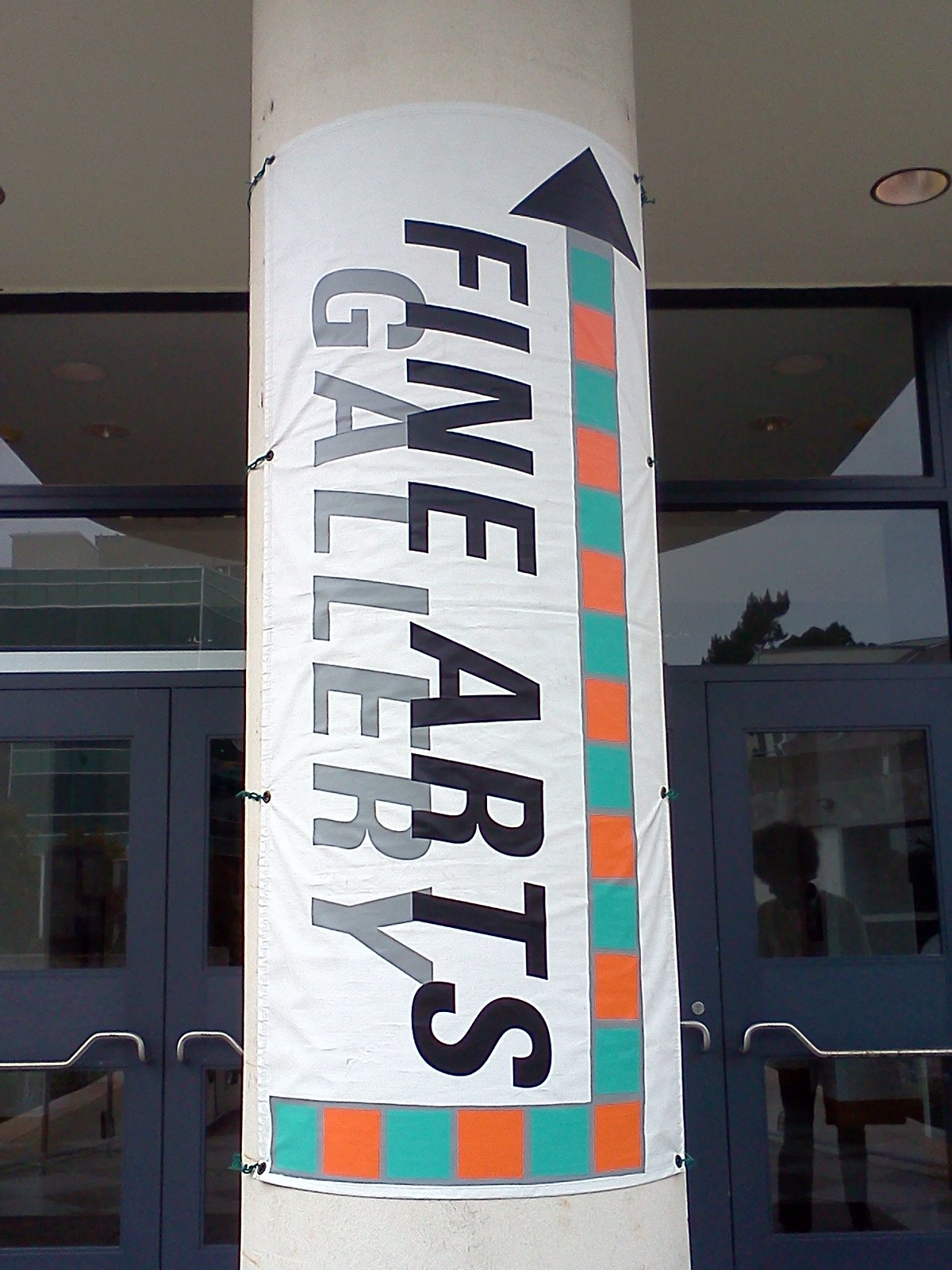The image depicts the entrance to a Fine Arts Gallery, marked by a large concrete pillar adorned with a predominantly white banner that reads "Fine Arts Gallery." The text "Fine Arts" is in black, while "Gallery" is in gray, accompanied by a green and orange multicolored arrow pointing towards the entrance. The entrance is framed by two sets of blue double doors with metal handles. Above the doors, the ceiling extends outward with a spotlight visible on the far right. The glass windows of the entrance reflect the surroundings, hinting at the bustling activity inside. Through the glass, a person with thick curly hair can be seen preparing to exit, casting a shadowy outline against the backdrop of the gallery's interior. The scene is a dynamic snapshot of this vibrant cultural space, inviting visitors to explore the fine art within.